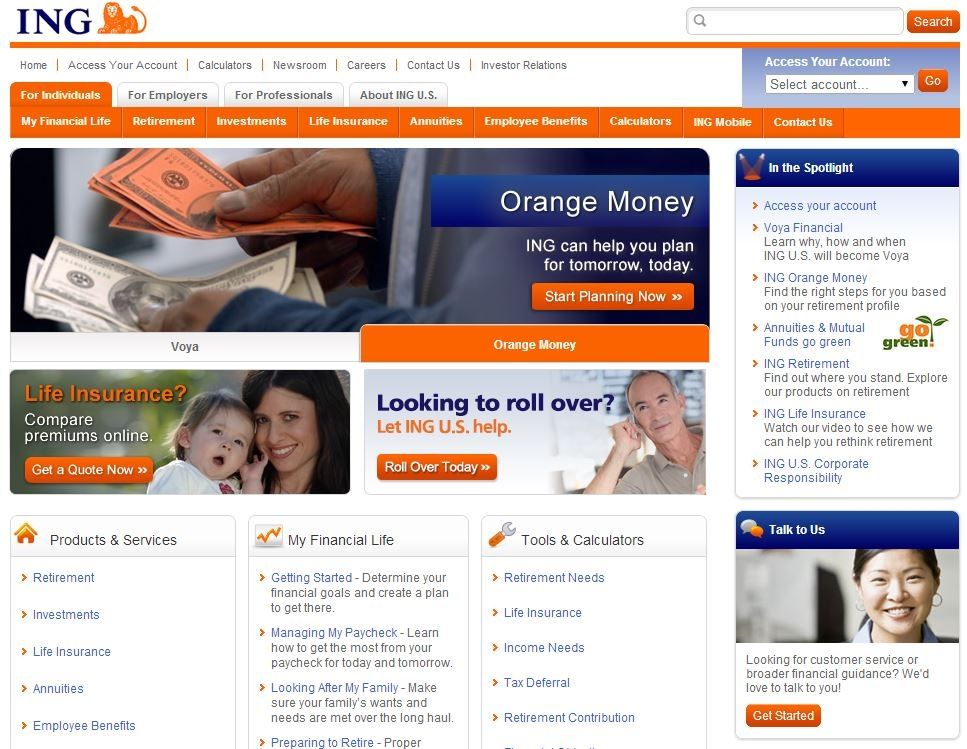A detailed screenshot of the ING homepage reveals key elements of their website's layout and features. At the top, the company's name is prominently displayed in bold black letters, accompanied by their signature orange lion logo, reinforcing their brand identity as a leading investment company. The background is predominantly white, lending a clean and professional look to the interface.

On the right-hand side, there's a search bar, equipped with a button to initiate a search after input. Directly below, a horizontal white navigation bar provides quick links to "Home," "Access Your Account," "Calculators," "Newsroom," "Careers," "Contact Us," and "Investor Relations." Further below, a series of tabs offer options tailored to different user categories—"For Individuals," "For Employers," "For Professionals," and information "About ING U.S."

Currently, the "For Individuals" tab is active, featuring comprehensive sections such as "My Financial Life," "Retirement," "Investments," "Life Insurance," "Annuities," "Employee Benefits," "Calculators," and a prominent "Contact Us" module. Above this section, a blue bar allows users to access their accounts directly by selecting the appropriate account type.

The main content area highlights ING's "Orange Money" concept, explaining how ING can assist in managing and planning finances. The illustration shows someone counting money, part of which is symbolically orange, emphasizing the brand’s color. To the right, a "Spotlight" section features various services and tools that users might find helpful. Additionally, the lower right corner includes an option for real-time communication, allowing users to easily get in touch with ING representatives. This layout underscores ING's commitment to providing comprehensive investment solutions and financial planning for the future.